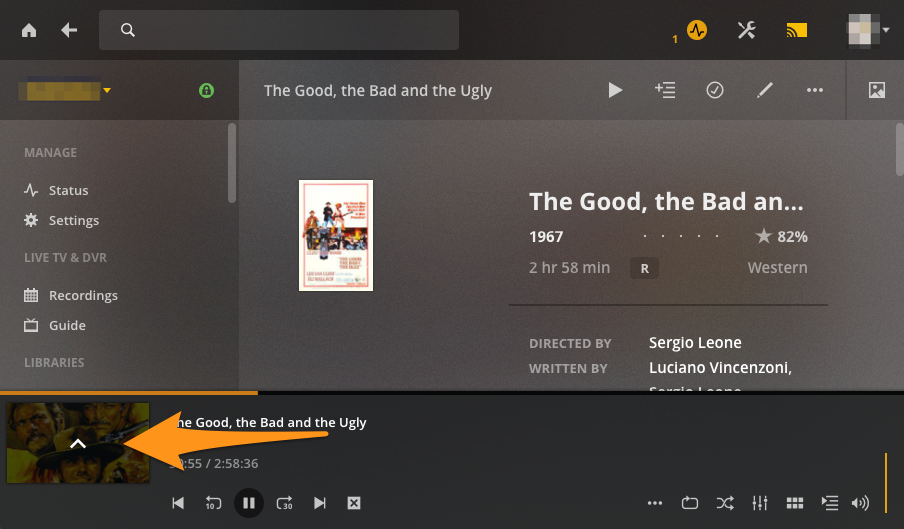A detailed screenshot of a video player interface, possibly a DVR or streaming service, featuring a mostly light gray and dark gray color scheme with some orange elements. The main focus of the image is a tutorial on how to resume a movie, highlighted by a large orange arrow pointing towards the thumbnail for "The Good, the Bad, and the Ugly." The thumbnail is accompanied by detailed information about the movie, including its duration, genre, star rating, director, and writer. In the upper right corner, account information and several icons are visible, such as a device casting option, tool settings, and a yellow squiggly line icon whose function is unclear. On the left side, a vertical navigation bar lists options like Manage, Status, Settings, Live TV and DVR, Recordings, Guide, and Libraries. At the bottom of the screen, a progress bar indicates that the movie has already been started, suggesting that the tutorial is demonstrating how to resume watching it.